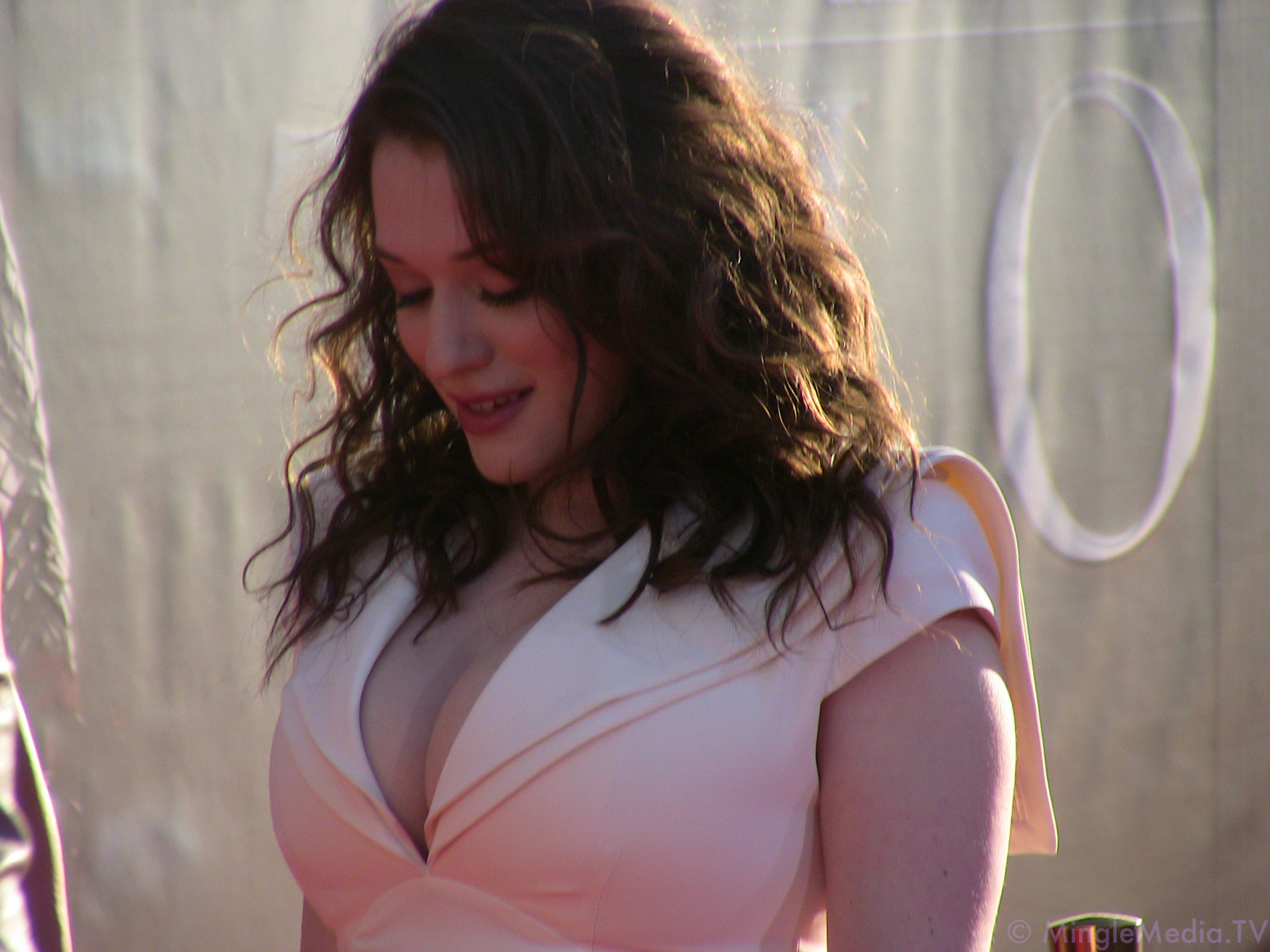The image features a young white woman, possibly a TV actress, posing for a head shot. She is wearing a seductive, creamy pink, low-cut dress that reveals part of her cleavage. Her brown, wavy, shoulder-length hair cascades down as she looks slightly downward with a subtle, half-smile on her face. Only her left arm is visible as she stands to the side. She is positioned against a light-colored wall, on which a white, raised letter 'O' can be seen, suggesting part of a word obscured by her head. In the bottom right corner of the image, a watermark displays, reading "minglemedia.tv."